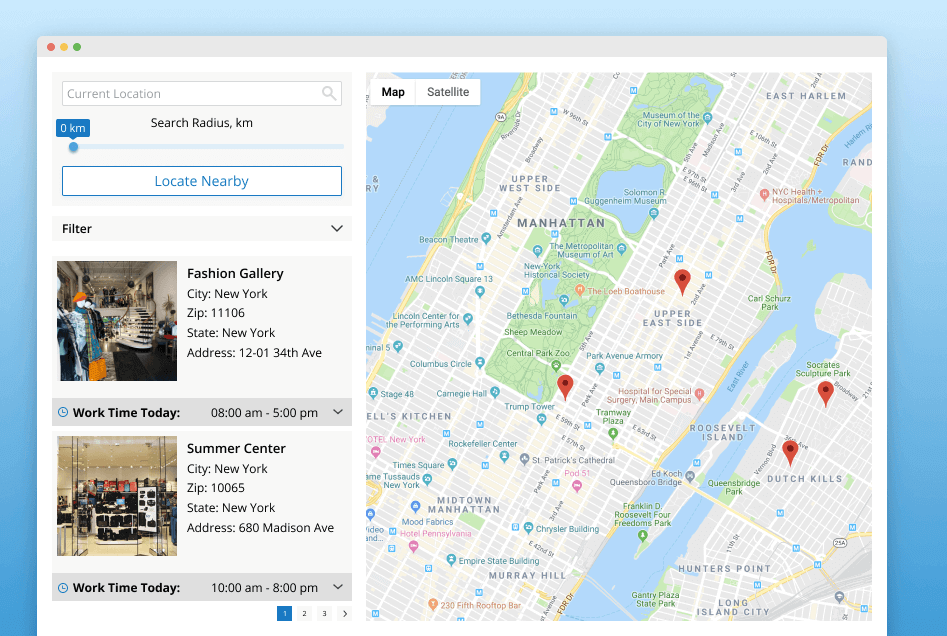**Detailed Caption:**

The image is a landscape-oriented screenshot from a website related to maps. It features a sky-blue border that extends across the top and down the left and right sides. The hue of the border varies slightly. Within this border, there is a main rectangular section that serves as the primary focus of the screenshot.

At the top of this rectangle, there is a light gray bar with three colored dots in the top left corner - red, yellow, and green - resembling a horizontal traffic light. Below this bar, on the left side, is a search bar that currently displays the text "current location" with a magnifying glass icon inside, indicating it is a search field.

To the right of the search bar is a street map of Manhattan, featuring Central Park prominently in the upper part. The map also includes locations such as Roosevelt Island, Dutch Hills, Long Island City, and various neighborhoods like Midtown, Upper West Side, and East Harlem. Four red location pins are visible: one in the Upper East Side, another near the southeastern corner of Central Park, one in Dutch Hills, and one in an unspecified park.

Beneath the search bar is a search radius slider set to zero kilometers by default, allowing adjustments to the search radius by sliding it to the right. Below the slider is a large button labeled "Locate Nearby." Further down, there is a black text label "Filter" accompanied by a drop-down menu.

Two search results are displayed beneath these filters. The first result is "Fashion Gallery," which includes a small square thumbnail image, its name, city (New York), state, address, and work hours (today from 8 AM to 5 PM). The second result is "Summer Center," also located in New York, with an address on Madison Avenue. The thumbnail image for this result suggests it is the interior of an upscale store, and its work hours are similarly specified.

Overall, the website appears to be an application designed to locate and provide information on various locations or businesses in a specific area.